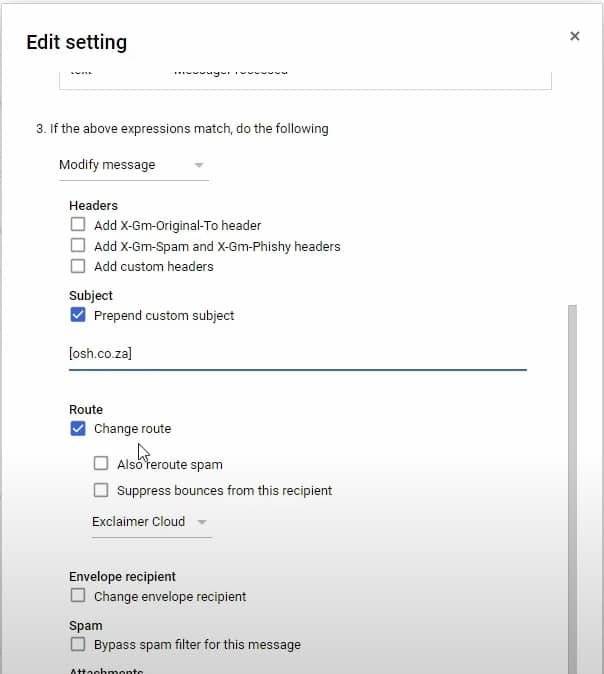The image is a screenshot focusing on an editing interface, which appears to be an email or message settings panel. At the very top of the interface, partially cut off, are the words "Edit Setting." On the top right corner, there is a small "X" button for exiting the interface.

The interface is scrolled down to the bottom, as indicated by the scrollbar positioned at the bottom right. The main portion of the window displays a series of detailed settings options, all presented in black text against a white background that gradually fades into gray towards the bottom.

At the visible top of this window is a numbered list item "3" which states: "If the above expressions match, do the following." This is followed by the directive "Modify message." Below this, a heading labeled "Headers" appears, with options to add three different headers.

Next, the caption describes a "Subject" section, featuring a checkbox labeled "Prepend custom subject," which is checked and highlighted in blue. The custom subject provided in this field is "osh.co.za" in brackets.

Further down, there is a "Route" section with a checkbox for "Change route," also checked and highlighted in blue. This section contains additional options: "Also reroute spam" and "Suppress bounces from this recipient," both of which are unchecked.

Following this, a heading labeled "Envelope Recipient" appears. Below this is another heading labeled "Spam," and partially visible below that, a heading titled "Attachments," indicating that there are more options available further down.

The interface layout is clean and minimalistic, with a gradient aesthetic that transitions from white at the top to gray at the bottom, providing a modern and functional design.